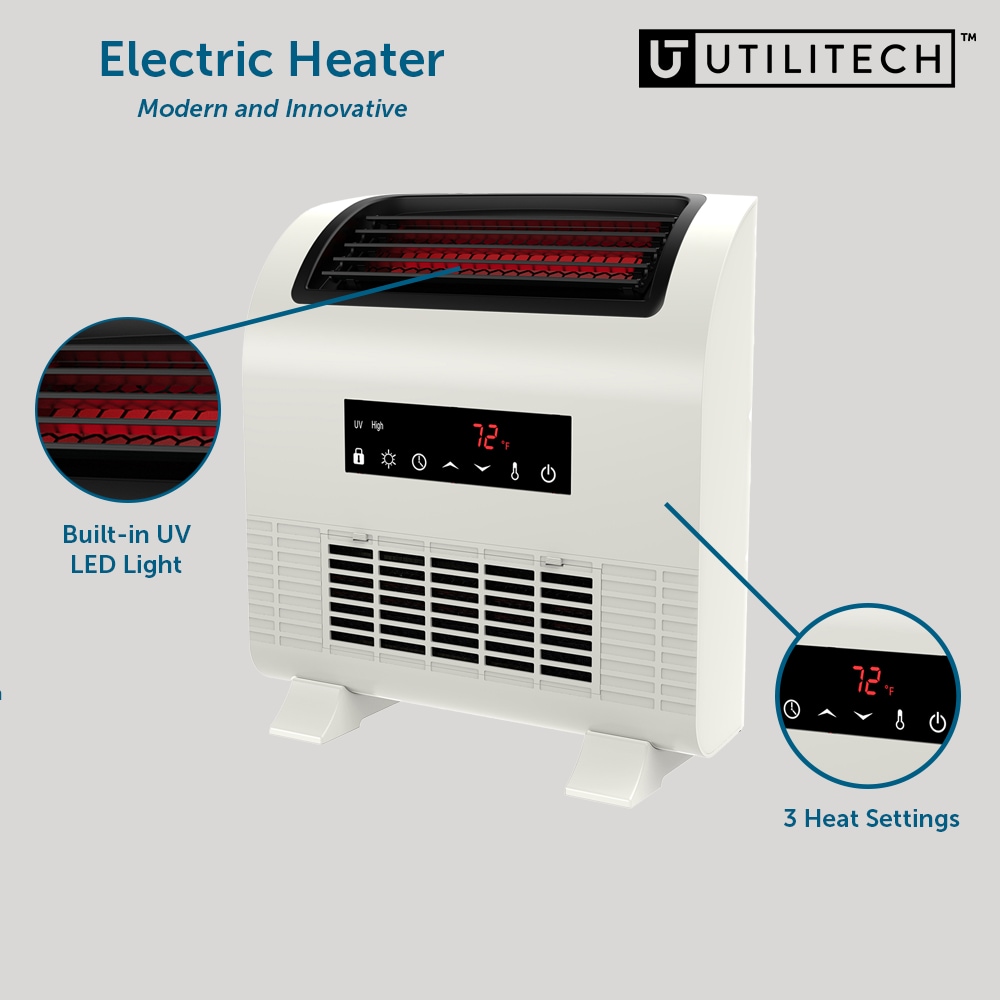The image depicts a modern, white electric heater with a unique, slightly curved, square shape. Prominently featured at the top is a black vent with glowing red coils indicating active heating. The top-left corner of the image has a caption in dark blue font that reads, "Electric heater, modern and innovative," and the top-right corner displays the brand name "Utilitech" in black lettering.

The heater stands upright, showcasing a sleek design with multiple noteworthy elements. In the center of the device, there is a small black LCD screen with various controls, including buttons for temperature adjustment, a lock, a timer, and a power-off button. The display shows a digital reading of 72 degrees Fahrenheit in red LED lights.

Additionally, there are descriptive callouts on both sides of the appliance. On the left, a bubble highlights the built-in UV LED light. On the right, another bubble emphasizes the three heat settings available. The overall background of the image is light gray, providing a clean and modern look to the advertisement.